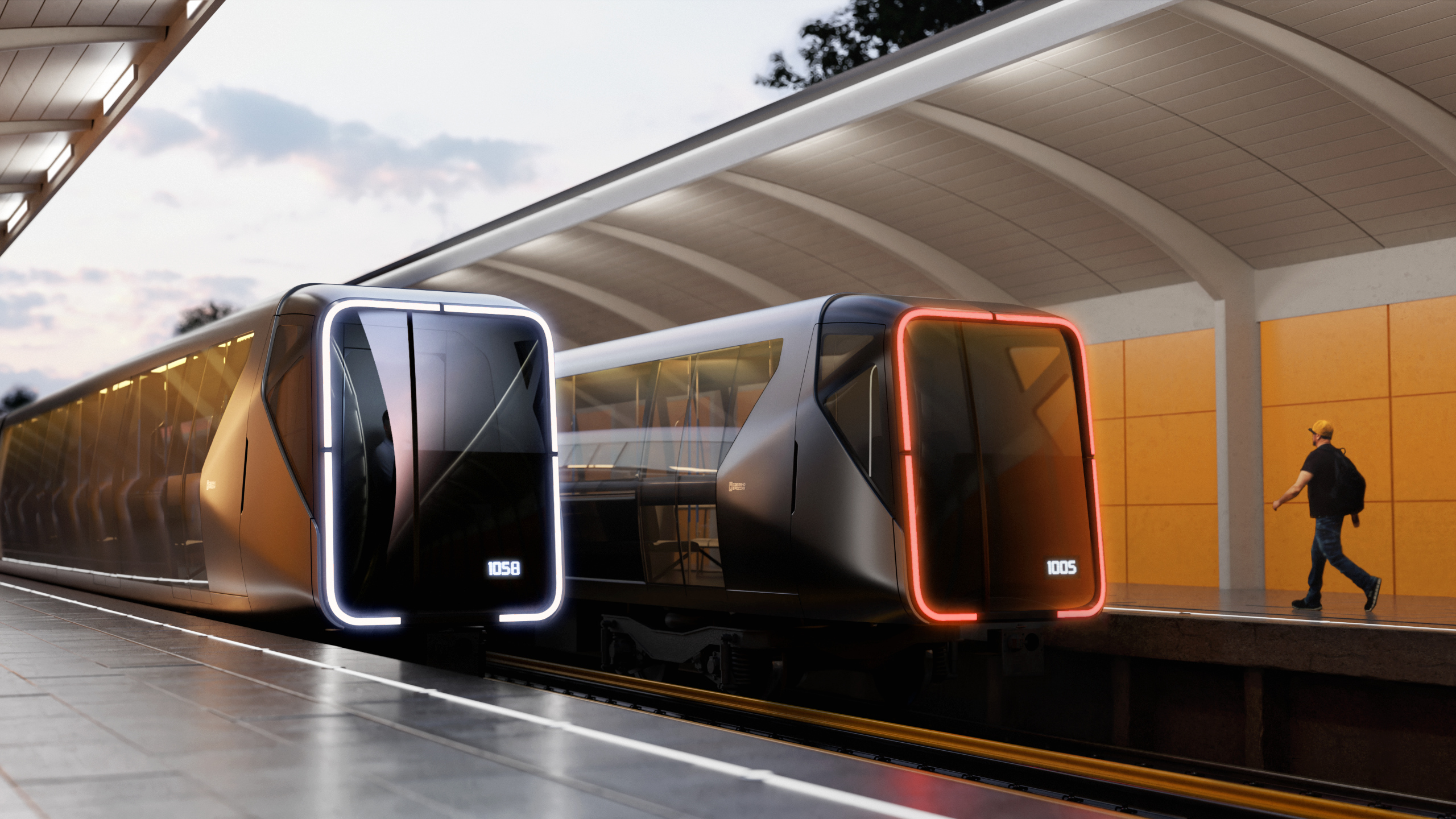The image captures a bustling train station terminal under a bright blue sky dotted with a few clouds. Dominating the scene are two modern, high-speed trains, both featuring a sleek, rectangular design with large windshields that form a bubbled, square-like shape at their fronts. These distinctive windshields are bordered by neon lights—white on the left train and red on the right—illuminating the respective trains which display digital numbers on their fronts: 1058 on the left and 1005 on the right. The trains, composed of a sleek gray and black color scheme, have clear and visible windows running along their sides. 

Between the two trains, the sky and the tops of some trees are visible through the gap, adding a touch of nature to the technological setting. The station features a gray floor marked with white safety lines, denoting safe distances from the trains. On the right side of the terminal, a bald man wearing a black t-shirt, blue pants, a backpack, and sunglasses strides along, set against an orange-lit wall. The trains are sheltered by a white overhang with a gray roof, mirrored on both sides of the station. The complex but symmetrical design of the terminal, combined with the vivid details of the trains and their surroundings, paints a vivid, dynamic picture of modern transit infrastructure.